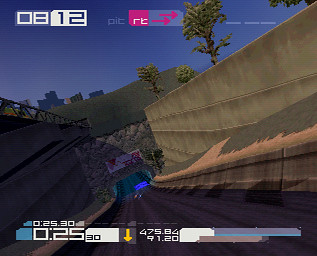This image captures a detailed scene from a computer game, depicting a road that leads downward into what appears to be the entrance of a city, situated underneath a subway or bridge. The setting is still outdoors, with the descending road transitioning into a well-illuminated area beneath the overpass. Flanking the road on either side are concrete structures, and the right-hand side is lined with trees, adding a touch of greenery to the urban environment. In the background, a cluster of skyscrapers reaches into the bright blue sky, indicating the presence of a bustling city. 

In the top left corner of the screen, a digital display shows "0812," likely indicating the time or an in-game metric. Adjacent to it, a sign reads "PIC RT," accompanied by two pink arrows pointing to the right, perhaps directing the player or providing an important in-game cue. At the bottom of the screen, several gauges and barometers provide additional information: one displays "02530," while another has a yellow arrow pointing downwards, contributing to the detailed and immersive gaming interface.